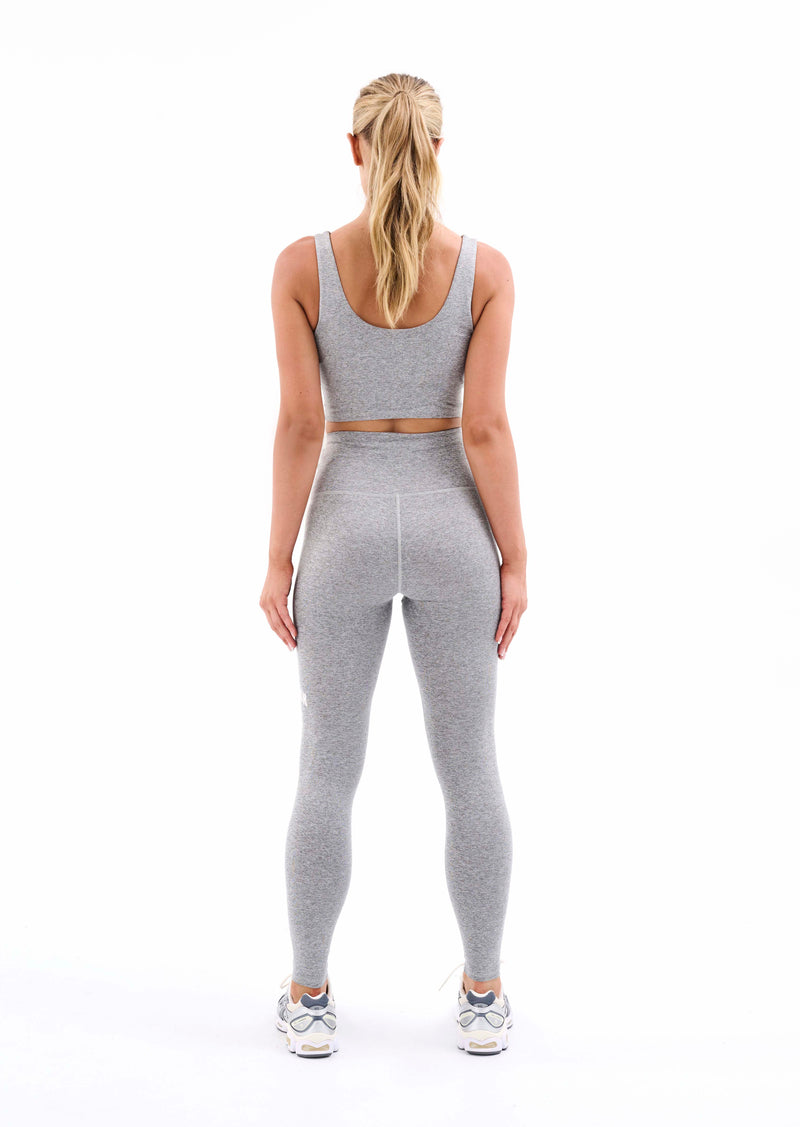This photograph showcases a young, fit woman standing in an exercise or yoga outfit against a stark white background, emphasizing her full figure centered in the frame. She is facing away from the camera, revealing her back but not her face. Her long, wavy blonde hair, with hints of brown at the roots, is pulled back into a ponytail that cascades down her neck. She is dressed in a coordinating heather gray ensemble, comprising a long sports bra or crop top that reveals a small inch of her lower back above her high-waisted yoga pants. Her white athletic shoes feature light blue accents, a matching sock insert with a dark blue rim, and darker blue soles. Her arms hang straight down by her sides, with her palms gently resting against her thighs, suggesting she is poised and ready to begin an exercise routine.